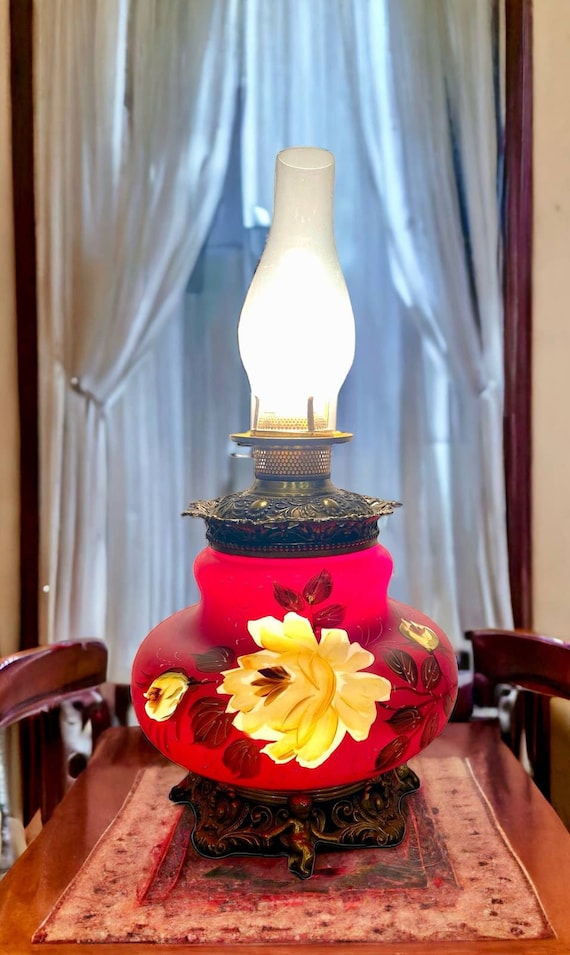This image depicts a detailed scene with a central focus on an intricate ornamental lamp placed on a polished, waxed wooden table. The lamp’s base is a vibrant red pot adorned with yellow flowers and reddish-brown leaves, giving it a glowing appearance. The wooden base of the lamp pot is decorated with carvings of playful cherubs. The lamp itself resembles a vintage, ornate gas or oil lamp, with a metal piece connecting the glass top to the glass vase-like pot. The lampshade starts wider at the bottom and tapers as it goes up. The table is covered with a decorative cloth in shades of pink, red, and black.

The background features a curtained window, possibly an entryway, with sheer curtains drawn to the sides. The overall scene includes additional indistinctively rendered furniture, suggesting an AI-generated composition. The details, such as the lack of discernible texture on the rug and the somewhat surreal quality of the window and furniture reflections, add to this impression.